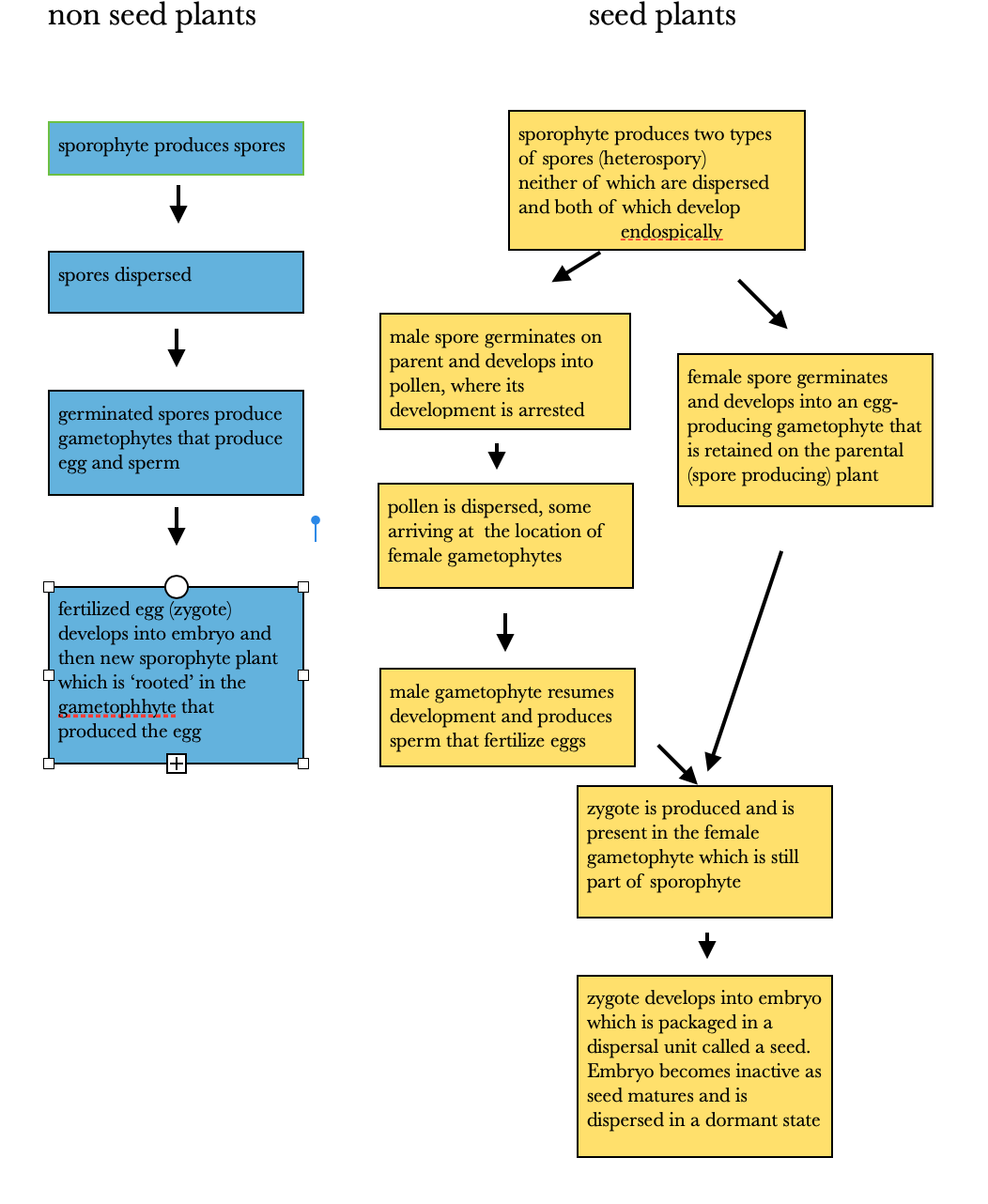This image presents a detailed flow chart contrasting the life cycles of non-seed plants and seed plants against a white background. The chart is divided into two columns: "Non-seed Plants" on the left with a sequence of blue boxes, and "Seed Plants" on the right with a series of yellow boxes.

In the "Non-seed Plants" column, the process begins with the sporophyte producing spores, which are then dispersed. The next stage involves germinated spores developing into gametophytes that produce egg and sperm. When fertilization occurs, the egg forms a zygote, which subsequently develops into an embryo and a new sporophyte plant, rooted in the gametophyte that produced the egg. Notably, there is a spelling error indicated by a red underline on the term "gametophyte."

In the "Seed Plants" column, the sporophyte produces two types of spores, both of which develop endosporically without being dispersed. The male spore germinates on the parent plant, forming pollen that, when dispersed, reaches the location of the female gametophytes. The male gametophyte then resumes development and produces sperm to fertilize the eggs. In a separate path, the female spore germinates and develops into an egg-producing gametophyte, retained on the sporophyte. The process concludes with the formation of a zygote within the female gametophyte, which remains part of the sporophyte. The zygote develops into an embryo, encapsulated in a seed. The embryo remains dormant as the seed matures and is eventually dispersed in this dormant state.